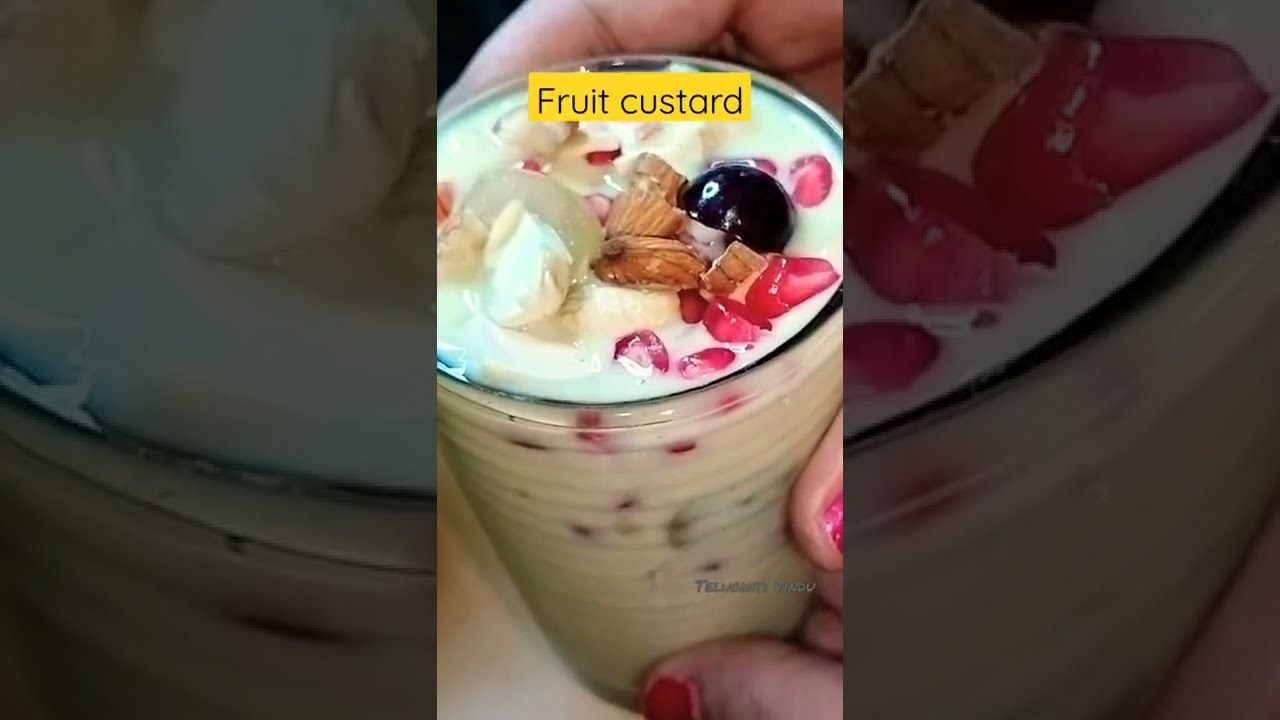The image is a close-up, high-definition photograph featuring a woman's hand, adorned with red nail polish, holding a glass cup of fruit custard. The glass has grooves along the sides, possibly for grip or design. The custard is predominantly white, suggesting a creamy base like yogurt or milk. On top of the custard, there are a variety of fresh toppings: visible almonds, a black cherry, pomegranate seeds, as well as slivers of other nuts such as walnuts. There are also berries, including a single blueberry and pieces of strawberries or raspberries. Clear, crystal-like ingredients add a unique texture and appearance. At the top of the image, there's a yellow caption in black font that reads "Fruit Custard." The image is divided into three parts, with the main photograph in the center and faded, close-up sections of the custard providing a darker, background border on either side, enhancing the focal point. The aspect ratio of the image suggests it may have been captured from a smartphone screenshot or video post, suitable for formats like Instagram or TikTok.